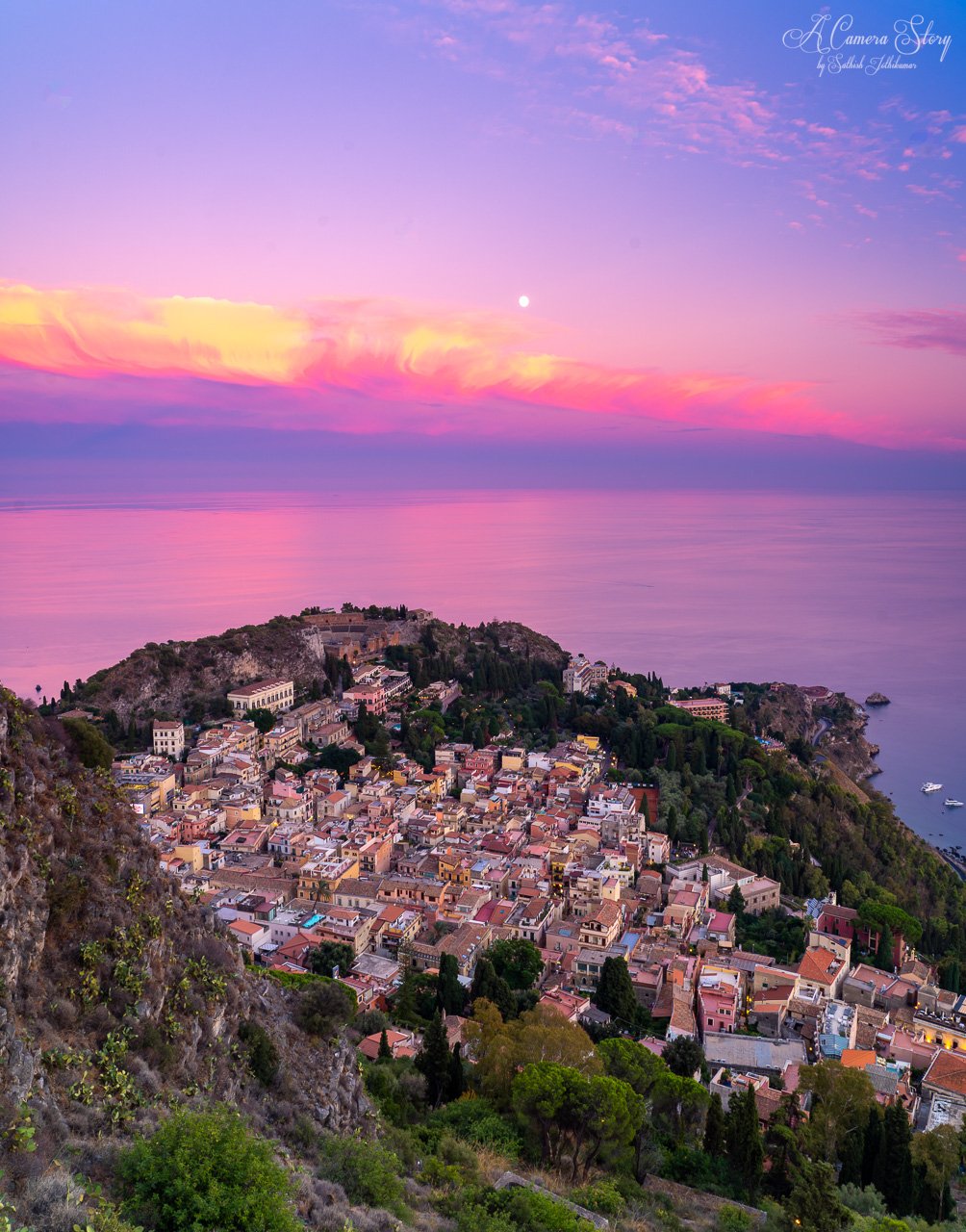The image captures an aerial perspective of a quaint, elevated village nestled within the natural barriers of a mountainous landscape. The village, consisting of colorful and charming one- or two-story buildings, is set against the breathtaking backdrop of a vast ocean. The scene is accompanied by a mesmerizing sky, painted in hues of orange, pink, purple, and golden as the sun sets or rises, casting its splendid colors over both the water and the village below. The ocean extends far into the distance, blending seamlessly with the sky, while the cliffs and green hills surrounding the village add to its picturesque allure. The setting feels like a potential tourist destination, possibly located in Italy or France, with hints of hotels near the water, inviting visitors to bask in its serene beauty.